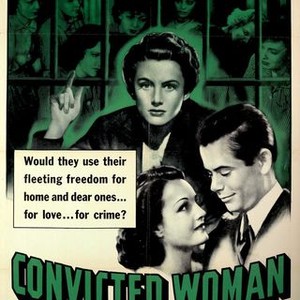The image appears to be a vintage movie poster or an advertisement for a show, with a stylized, old-fashioned aesthetic. The top half of the poster features a dark green background with green jail cell bars, behind which stand around eight women. Prominently in the foreground, a gray-skinned woman with black hair, possibly a lawyer given her attire—a collared shirt and suit jacket—is pointing towards the background, her intense expression aimed directly at the viewer. Below this, the bottom half of the poster transitions to a more congenial scene in black and white, depicting a young couple, likely in their late 20s or early 30s, smiling warmly at each other. The man, clad in a tie, sweater vest, and collared shirt, looks lovingly down at the woman, who beams up at him, suggesting a deep emotional connection. Superimposed on this lower half, the title "Convicted Woman" appears in bold green block letters. To the right, a text bubble reads, "Would they use their fleeting freedom for home and dear ones, for love, for crime?" further adding to the intrigue of the narrative being conveyed.